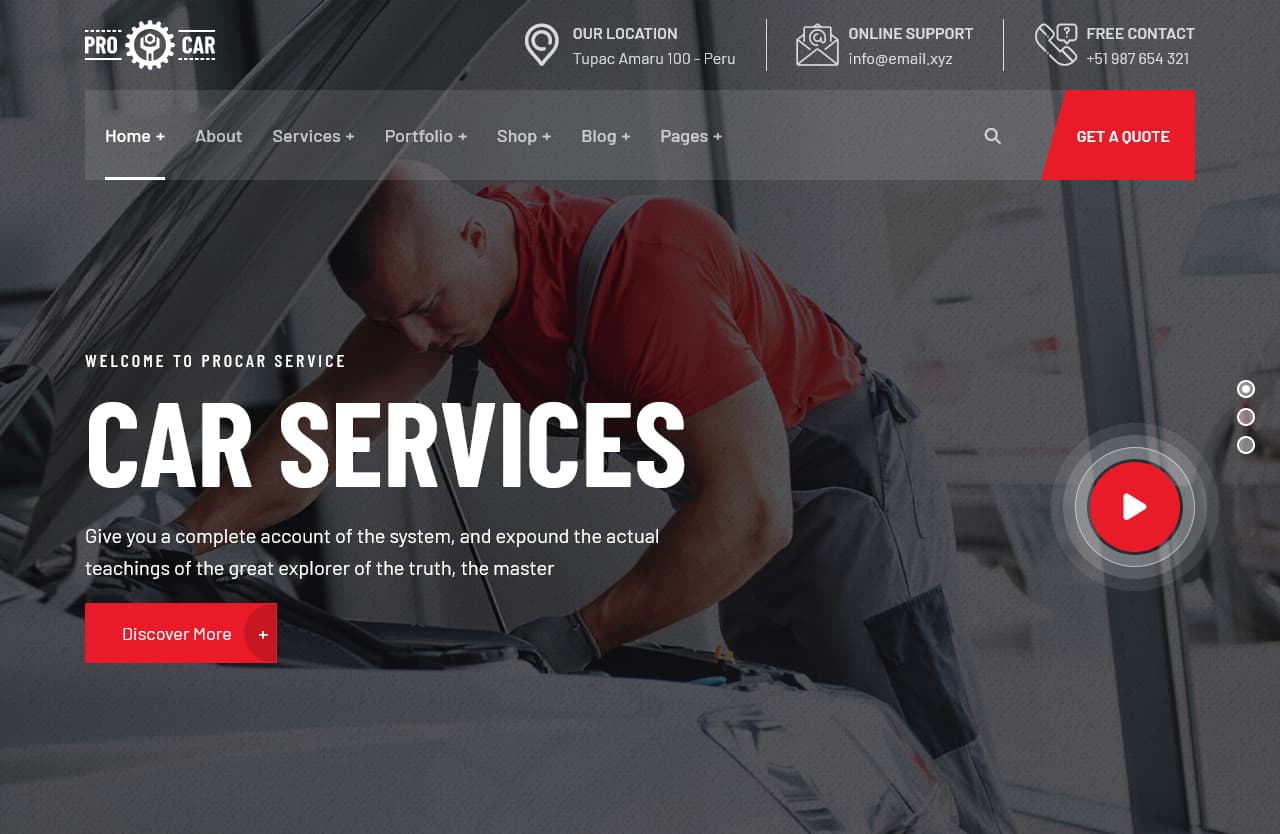In this image, we see what appears to be a screenshot of a webpage featuring an almost black-and-white background with subtle yet noticeable elements. Central to the image is a Caucasian man of European descent, seemingly a mechanic, engaged in work under the hood of a white car. He is dressed in gray overalls, gray gloves, and a red shirt, and has a shaved head. His arms are extended into the car engine, indicating he is performing some sort of technical task.

At the top-left corner of the image, there is a white emblem resembling a cogwheel, next to the word "Pro" in bold. Adjacent to this, the word "Car" is displayed. Below this, a semi-transparent gray banner contains a navigation menu with drop-down boxes labeled "Home," "About," "Services," "Portfolio," "Shop," "Blog," and "Pages." To the right of this banner, there's a magnifying glass icon indicating a search function. In the middle of the white backdrop, there's a prominent call-to-action button that reads "Get a Quote" in red text.

Above the banner, in white font, is location information stating "Our Location: Tupac Amaru 100, Peru," followed by vertical divider lines. Next, symbols for email and phone support are present. It reads "Online Support: info@example.com" and "Free Contact: (123) 456-7890" alongside respective icons resembling an envelope for email and a chat bubble with a question mark for phone support.

Just below the man's face, there is a welcoming message in small white font that says, "Welcome to Pro Car Service." This is followed by a larger white font displaying "Car Services." In very small print, the text continues, "Give you a complete account of the system, and expound the actual teachings of the great explorer of truth, the master." Beneath this text, there is a small red drop-down box with white text that reads "Discover More" accompanied by a plus sign.

To the right of this section, there is a circular play button in red, akin to a YouTube play button, featuring a white triangle in its center, suggesting it can be clicked to view a video. The overall composition suggests a professional automotive service website, providing detailed information and call-to-action elements to engage visitors.